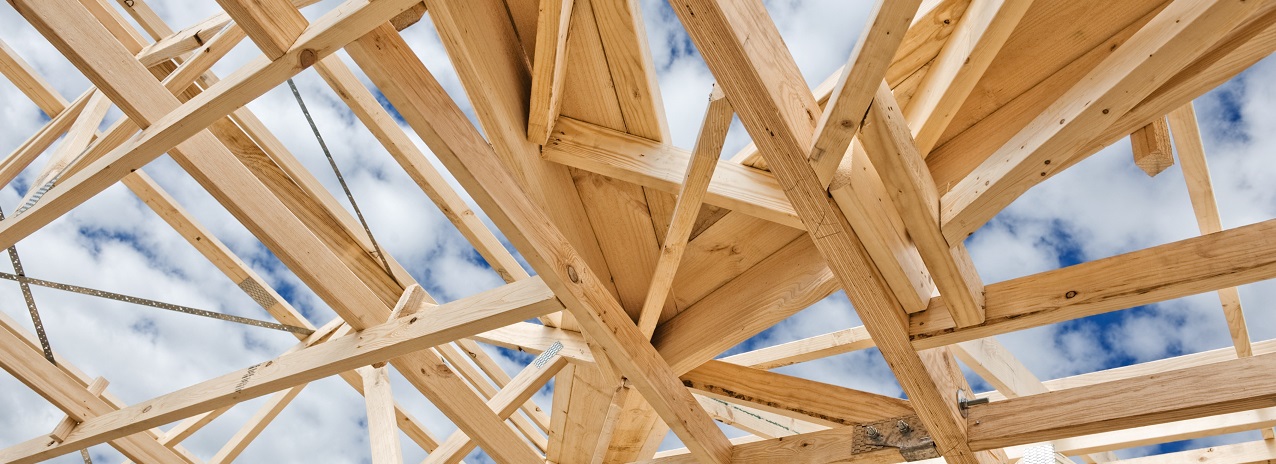This color photograph, taken from below, captures the intricate framework of an unfinished building, looking upwards towards a predominantly cloudy blue sky. The image showcases a complex arrangement of light brown wooden beams and boards, some showing knot holes, creating an open roof structure. These wooden elements, resembling 2x4s, are nailed together in different lengths and shapes, forming trusses and braces that stretch in various directions. The beams run diagonally, horizontally, and vertically, resulting in a dynamic, crisscross pattern with noticeable gaps that allow the sky, covered 80% by white fluffy clouds, to be visible. The chaotic, yet methodically connected beams highlight the ongoing construction, where the interplay of sky and wood frames a scene of architectural progress.